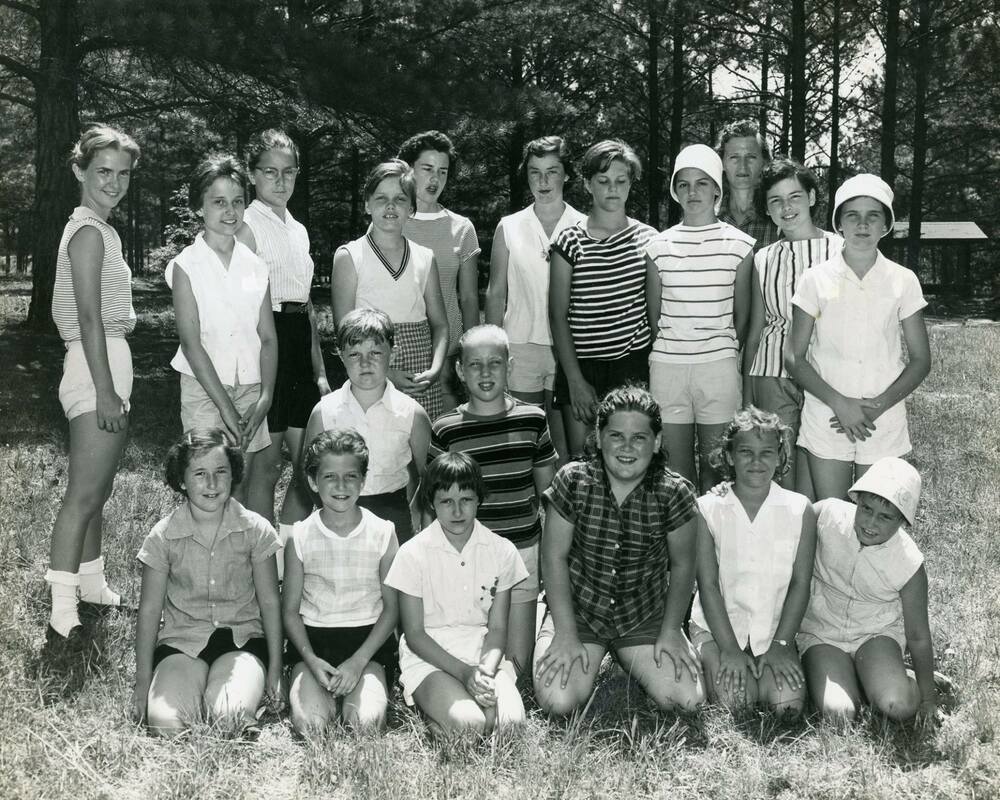This is a black-and-white photograph depicting a summer camp scene from the 1950s or 60s, featuring a group of predominantly white, suburban children aged between 10 and 15. The kids are arrayed in rows on a field of grass, with the front and middle rows kneeling while the back row stands. Most of the children are wearing short-sleeved white shirts, very short shorts, white socks, and black shoes. Some wear white caps, and one child is notably dressed in a black-and-white striped shirt, while another sports a plaid shirt and appears larger even while kneeling. Among the kids, there’s a perplexing figure donning a lampshade on their head. A child with a receding hairline, unusually prominent for their age, also stands out. Several of the girls are dressed in v-neck shirts and some striped patterns. The backdrop features a dense forest with pine trees and a cabin, suggesting the setting is deep in the woods, far from suburban houses. All the kids are smiling, capturing a joyous moment frozen in time.